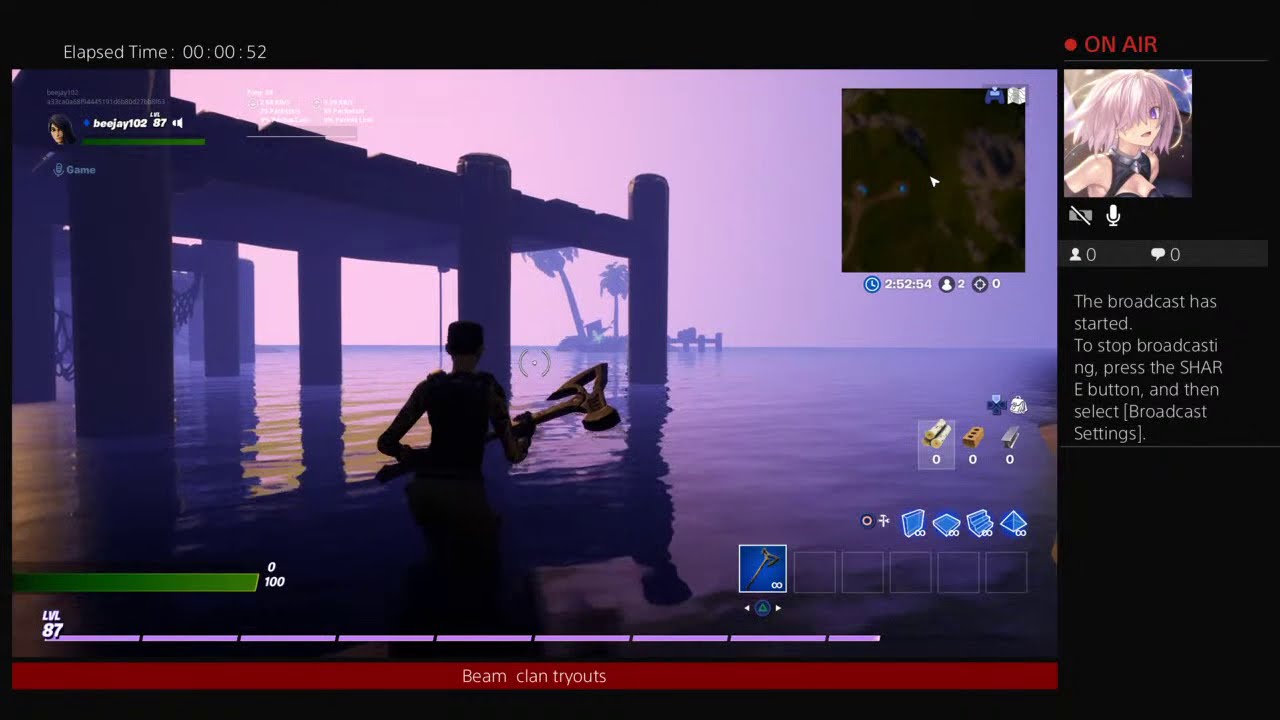The image is a detailed screenshot of a video game, which appears to be streaming live. Central to the image is a gameplay scene, set against a backdrop of a purplish-pink sunset. A character, wading through waist-deep water, faces away from us while holding a large axe. The character, whose gender is ambiguous but leans towards female based on the shape, stands near a tall pier. In the distance, there is a small island with a couple of palm trees. The water and sky are infused in hues of purple and blue, suggesting an evening setting.

Surrounding the gameplay are various broadcasting details. In the top left corner, a timer counts elapsed time at 00:00:52. The top right corner features a map, and to the right side, written in red letters, it says "On Air." Below this text, there is a profile picture of an anime girl with pink hair and a corset outfit. Indicators beside the profile show zero viewers and zero comments; icons here include a bright microphone symbol and a dull gray camera-off symbol. Below, white text reads, "The broadcast has started. To stop broadcasting, press the Share button and then select Broadcast Settings."

At the bottom of the screen, a red horizontal banner displays the words "Beam Clan Tryouts" in white text. Alongside, on the bottom left, there's a green health bar showing 100, and to the right, a segmented purple bar indicating the player's level at 87, nearly reaching 88. The player's inventory, featuring the axe and other items, is also visible here.